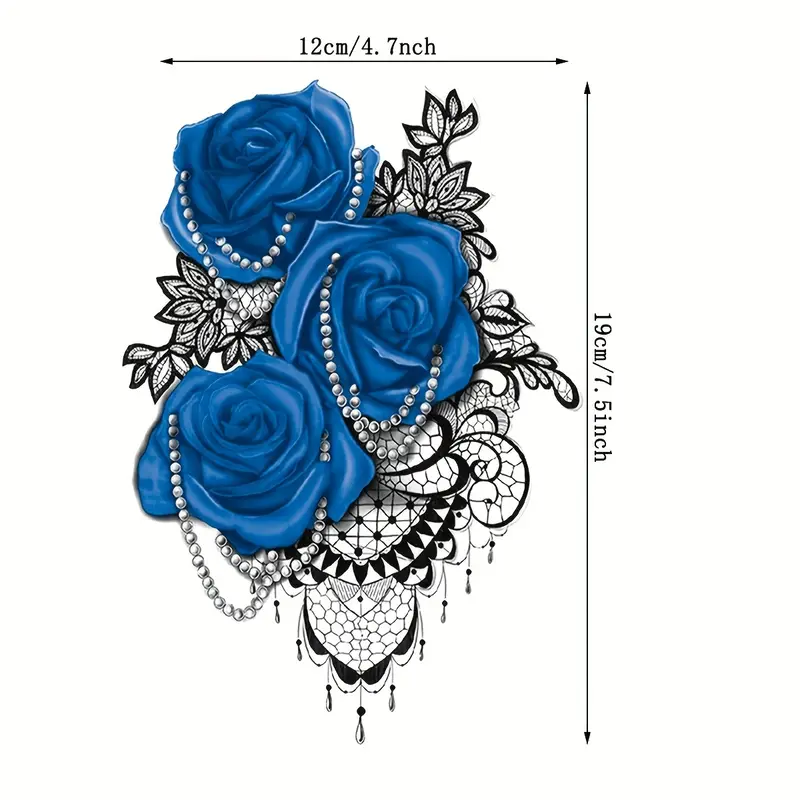A detailed black-and-white drawing designed for a potential tattoo showcases intricate details and precise measurements. The centerpiece features three vividly blue roses, each adorned with delicate white pearl necklaces. The pearls are intricately wrapped around the petals, with the top rose having pearls looped underneath and the second rose displaying two visible loops of pearls. The bottom rose has pearls elegantly draped around and hanging down. Surrounding the blue roses is an elaborate black and white filigree pattern that resembles lace, with delicate leaves and tassels adding to the complexity of the design. In addition, a measurement marker is included at the top, indicating the width of the tattoo as 12 centimeters (4.7 inches) and the height as 19 centimeters (7.5 inches). The width marker includes an arrow pointing left and right, while the height marker features a vertical line with arrows at both ends pointing up and down. This beautifully detailed composition merges the elegance of the blue roses and pearls with the classic sophistication of the black-and-white lace background, making it a striking tattoo design.